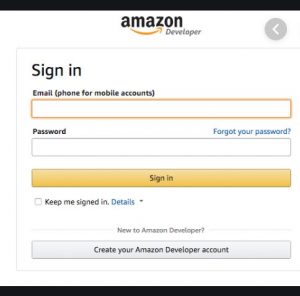In the image, we are viewing an Amazon website page, specifically the Amazon Developer sign-in page. The layout features distinct black horizontal borders along the top and bottom edges. The background is predominantly white, creating a clean and modern aesthetic.

At the center of the page, just below the top black border, is the Amazon Developer logo. The word "Amazon" is prominently displayed in bold black text, with "developer" in smaller black text directly beneath it. Adding to the iconic brand look, the familiar yellow arrow underlines the word "Amazon." To the right of this logo, there is a circular icon featuring a left-pointing arrow.

Below this section, a light gray border frames a white rectangular sign-in box. On the top left corner of this box, "Sign-In" is presented in bold black text. Directly below, there is a highlighted yellow input field labeled "Email (phone for mobile accounts)." Beneath this, another input field is present for entering the password.

Overall, the page is designed with simplicity and functionality in mind, ensuring an intuitive user experience for those signing into the Amazon Developer account.